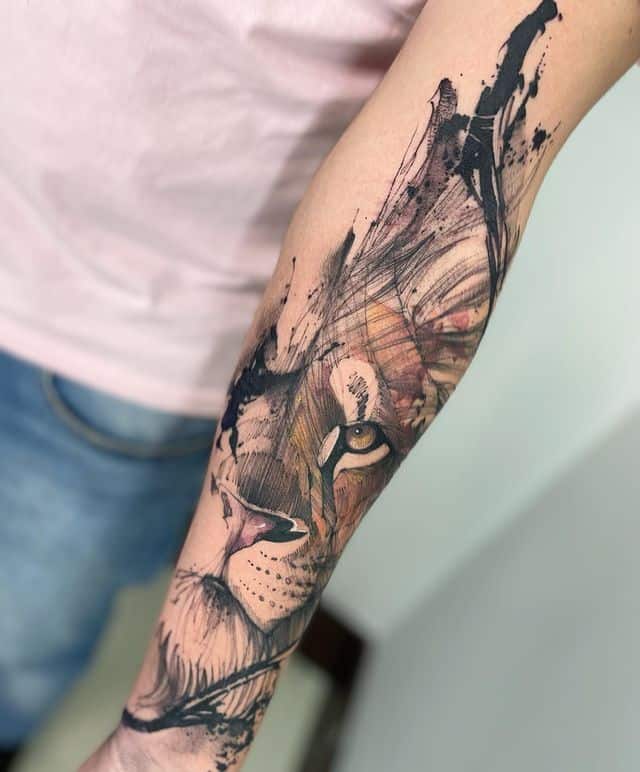The image displays a detailed, colorful tattoo on the arm of a woman with light skin. The primary focus of the tattoo is a lion's face, rendered meticulously, with the right side more developed. The lion's eye on this side appears to be looking directly at the viewer, creating a sense of interaction. The nose is finely detailed and painted pink, while the fur of the mane is indicated below it. Above the lion's head, instead of traditional ears, the tattoo artist has employed an artistic technique that incorporates paint splatters, allowing the viewer to use their imagination to fill in the gaps, contributing to an intentionally smudged and unfinished look. The tattoo features a palette of black, gold, pink, and hints of purple. The woman in the image is wearing jeans paired with a pink top.